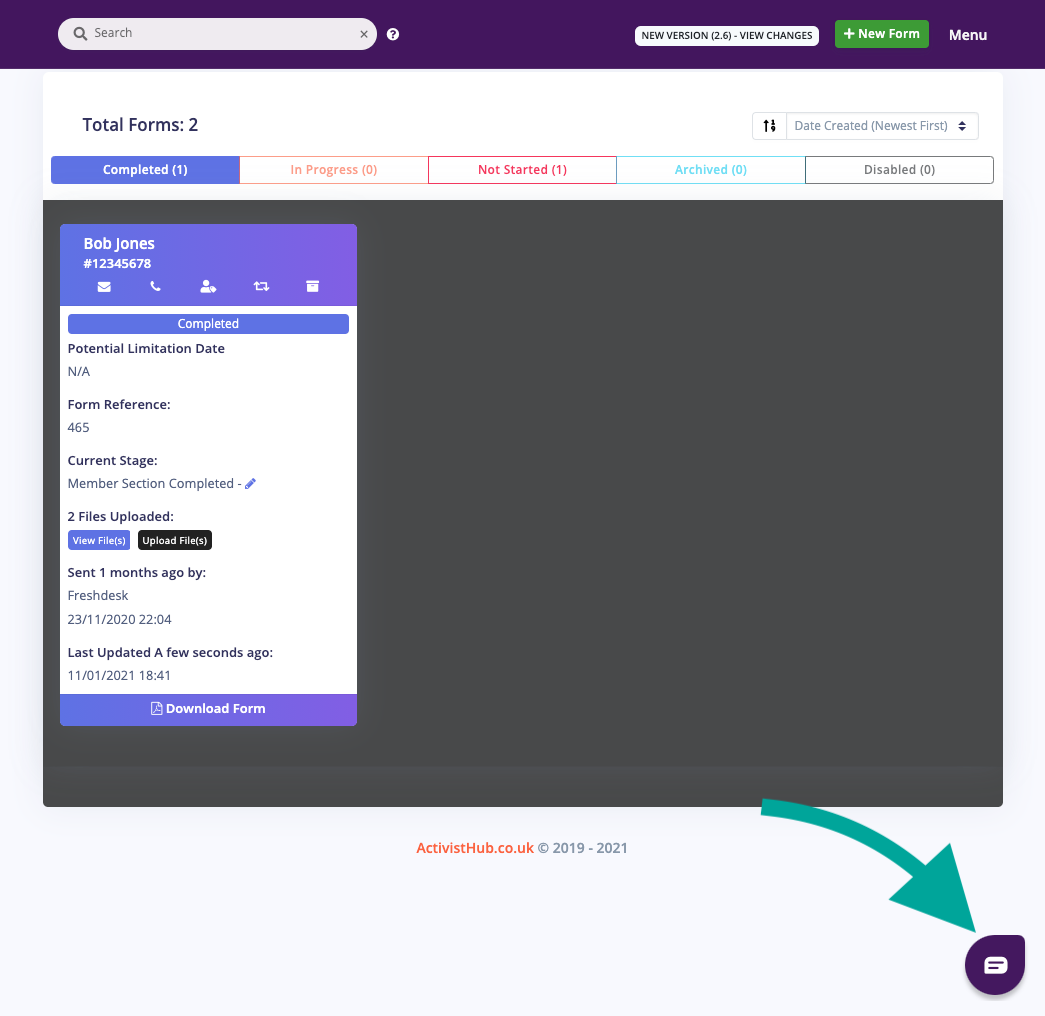The image captures a computer screen displaying a website. At the top of the screen is a purple rectangular header featuring a white search bar and a white question mark icon. There is a notification indicating "New Version 2.6" with an option to "View Changes." The header also includes a "New Form" section labeled as a "Menu."

Below this header, the screen displays various content. Toward the bottom, a teal arrow points towards a speech bubble icon within a purple, teardrop-shaped circle. The website footer reads "activisthub.co.uk © 2019-2021." Additionally, in the center of the screen, there is a periwinkle-colored rectangular section.